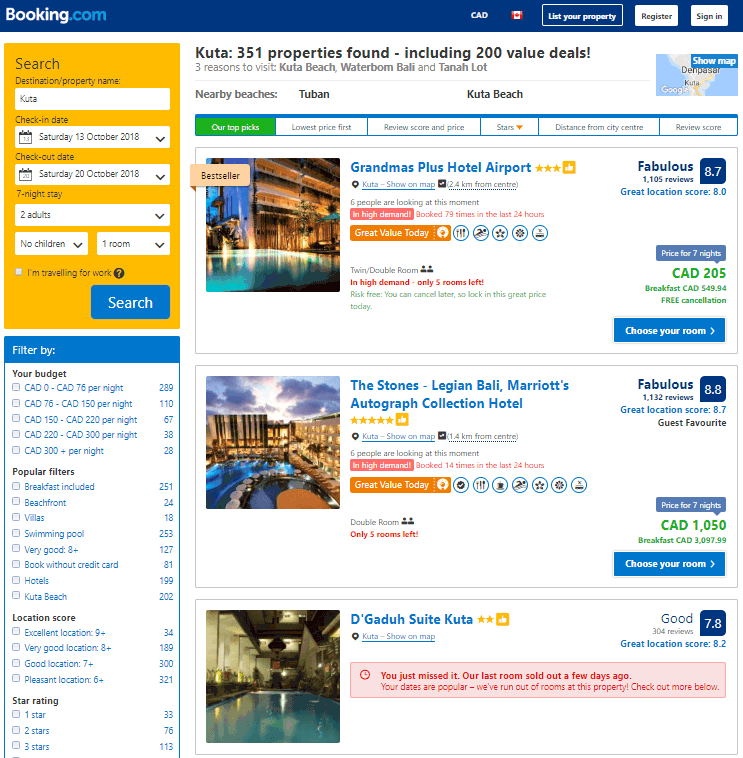This is a screenshot of the Booking.com website. The logo is prominently displayed in the top left corner, featuring "booking" in white text and ".com" in blue text, all set against a dark blue header. On the right side of this header, there are buttons for "Sign In" and "Register."

Beneath the header, there is a yellow search bar, indicating a booking query for Kuta. The check-in date is listed as Saturday, October 13, 2018, and the check-out date is Saturday, October 20, 2018, indicating a seven-night stay. The search specifies accommodation for two adults, no children, and one room.

At the bottom right of the search bar, there is a dark blue button labeled "Search." It appears that a search has already been performed, as search results are visible in the bottom portion of the screenshot.